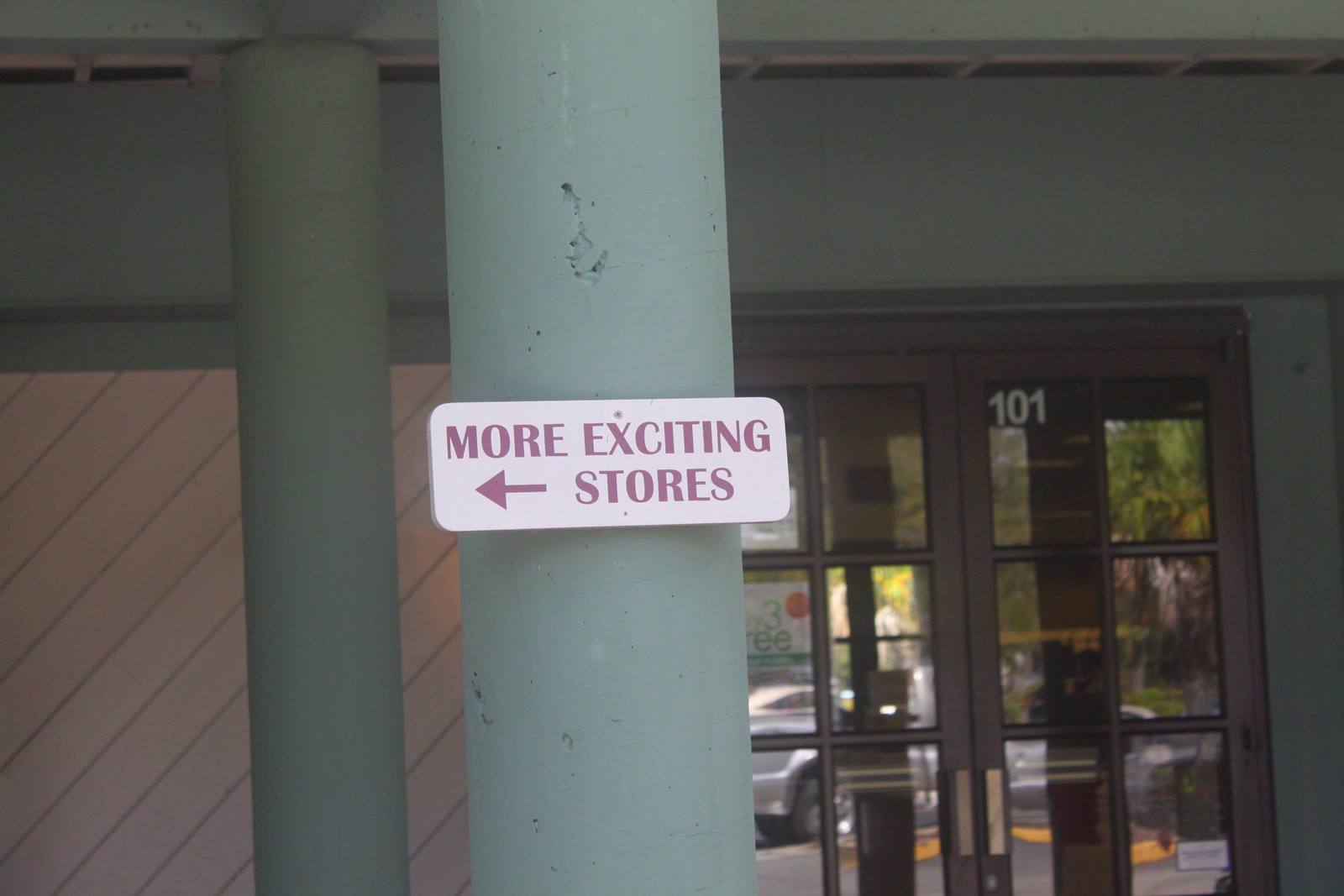This photograph captures a white, rectangular sign with rounded edges mounted on a green cement pillar outside a building. The sign features capitalized text in a pinkish-red hue that reads "MORE EXCITING STORES" with an arrow pointing to the left. Behind the primary pillar, another identical pillar is visible. The building’s exterior wall is adorned with wooden panels, adding a rustic charm. Two black-framed doors with nine glass panels each are also present, blending seamlessly with the setting.